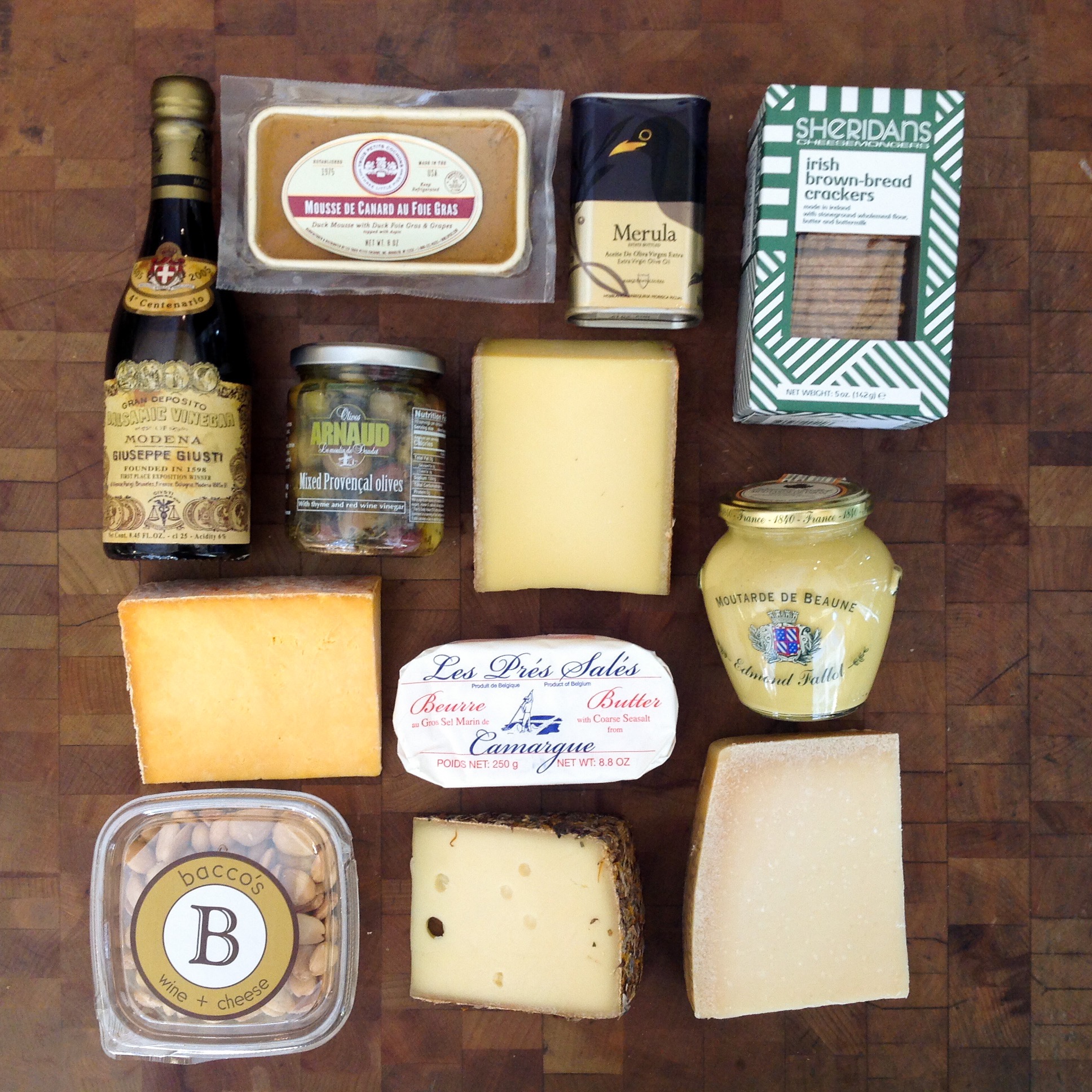The image presents an exquisite arrangement of high-class snack items meticulously placed on a dark brown wooden surface. The items form an almost grid-like pattern, enhancing the visual appeal and accessibility. Among the array, several wedges of high-quality cheese with rinds are prominently displayed, including a darker yellow cheese, a very light-colored one, and a white cheese wrapped in French-labeled white paper. Accompanying the cheeses, there is a vintage-looking bottle of wine with a brownish label, a dark bottle of balsamic vinegar with an old beige label, and a jar of Dijon mustard. Enhancing the gourmet experience, there is a plastic package of prosciutto or ham, a box of pistachios, and a tin can labeled 'marula.' Completing the spread are French butter wrapped in white packaging with blue and red lettering, a box of Sheridan's Irish Brown Bread Crackers, a small jar of olives, a square package of foie gras in clear packaging, and a plastic container labeled 'Bacos' with a large letter 'B'. Each item is carefully positioned, ensuring that their labels and details are clearly visible against the backdrop of the richly textured wooden blocks.